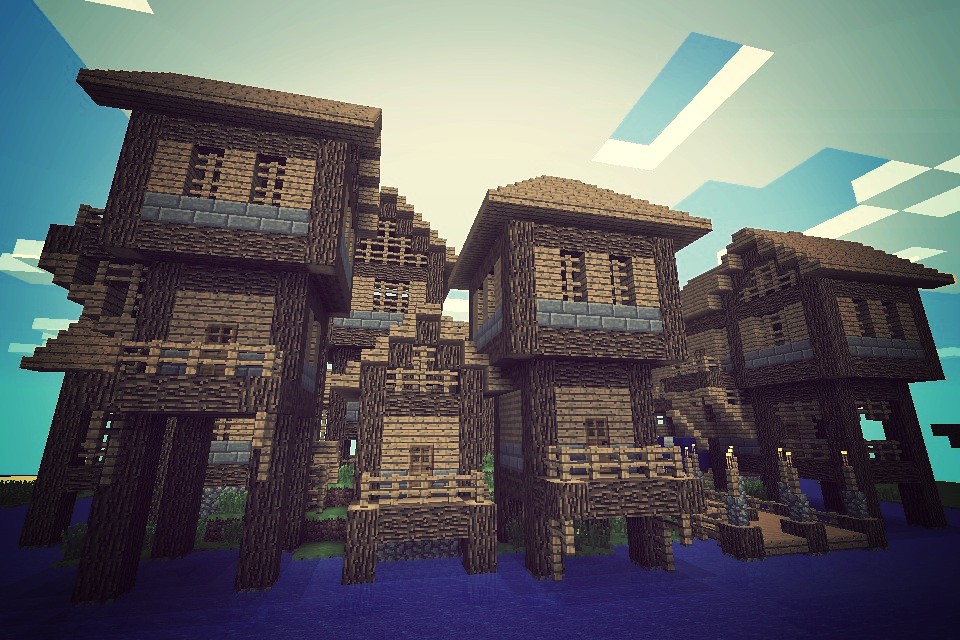This is a highly detailed, computer-generated image from the game Minecraft. The scene showcases a cluster of five intricately designed buildings made predominantly of wood and brick. Each structure displays a layered texture and depth, with uniformly brown roofs, dark brown edging around tall windows, and light brown wooden decks reminiscent of porches or balconies. The image includes stone columns capped with bright yellow lights, adding to the architectural variety. Surrounding the buildings are green shrubs and blue water, under a sky filled with clouds. The buildings have small windows and gray brick ledges across their fronts. Some structures exhibit multiple floors with wooden fences and torches on the right side, emphasizing their detailed craftsmanship within the pixelated aesthetics of Minecraft.